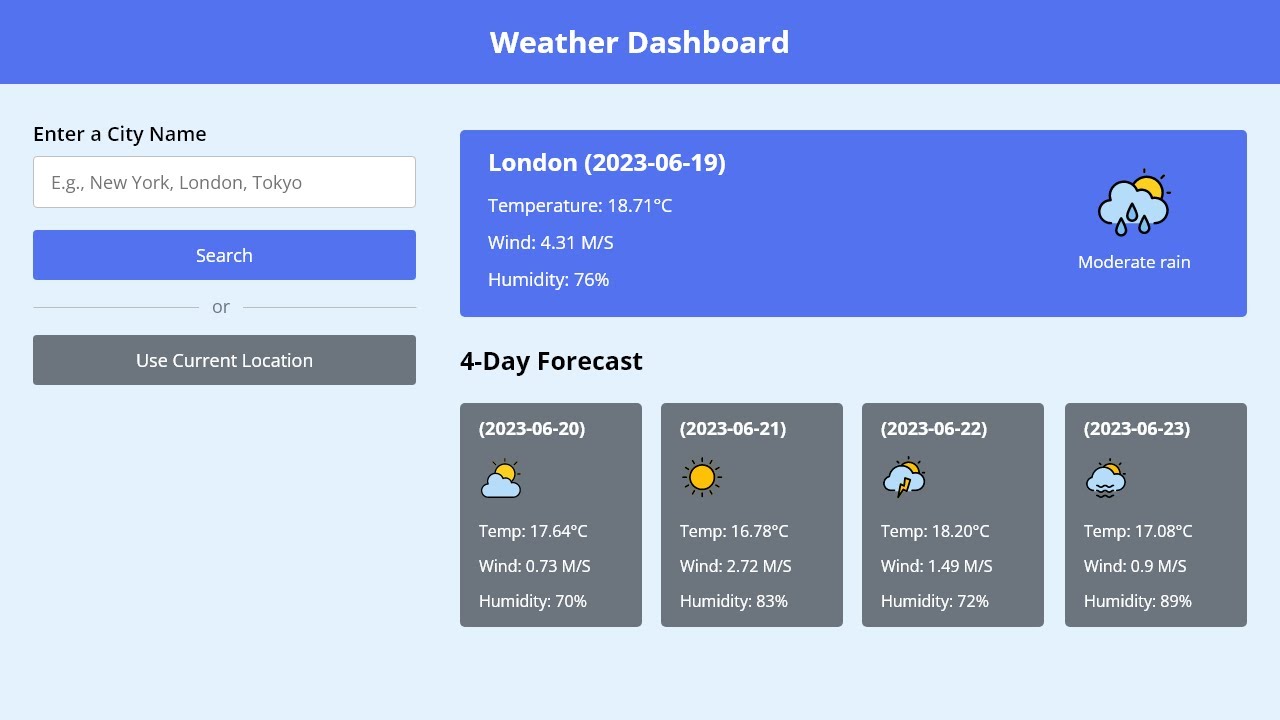In this image, there is a detailed screenshot of a weather dashboard application. At the very top, a dark blue rectangular banner displays the title "Weather Dashboard" in bold, white text. Below this banner, the background transitions to a light blue color.

On the left side of the screen, there is an input section prompting the user to "Enter a city name." This section includes a text box pre-filled with suggested city names: "New York, London, Tokyo." Beneath the text box, a blue "Search" button is prominently displayed. Below the search button, a gray divider line separates the input options, with the word "or" written on the line. Beneath this line, there is a gray button labeled "Use Current Location."

On the right side of the screen, information about London's current weather and forecasts is presented. The data indicates:
- Location and Date: "London, 2023-06-19"
- Temperature: "18.71°C"
- Wind Speed: "4.31 m/s"
- Humidity: "76%"

Below this weather summary, the section titled "Four Day Forecast" provides weather predictions for the upcoming days. Each day is represented by its date and a corresponding weather icon:
- June 20: Partly cloudy with some sun
- June 21: Sunny
- June 22: Stormy
- June 23: Rainy

This organized layout presents a comprehensive weather overview, blending user interactivity with detailed meteorological data.